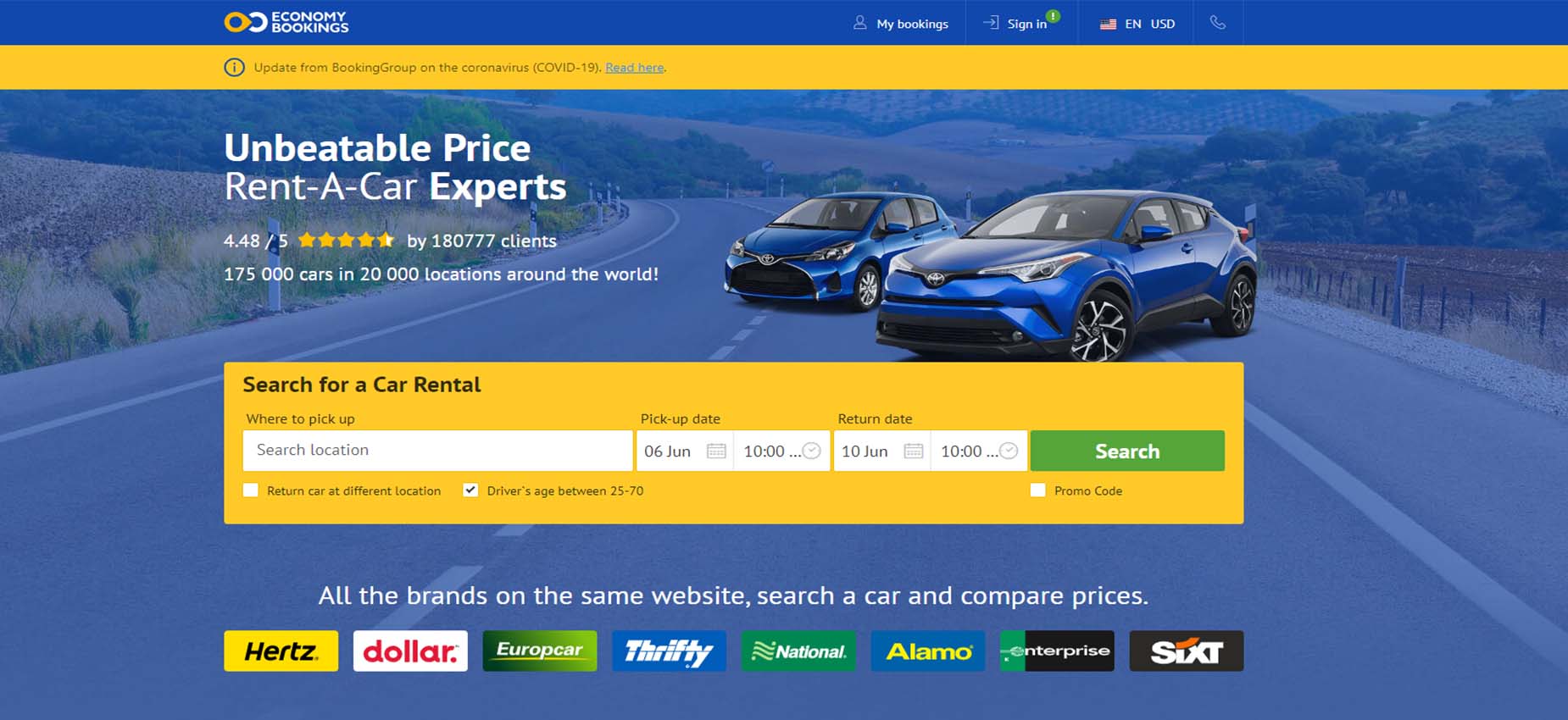This screenshot captures a car rental service website designed with a predominantly blue and yellow color scheme. The website features a vibrant blue header bar displaying the text "Economy Bookings" alongside a logo resembling a figure-eight, where the left section is orange and the right section is white. The name "Economy Bookings" is stacked below the logo. To the right of the logo, navigation options include "My Bookings," "Sign In," an American flag icon indicating English language and U.S. dollar currency, and a phone receiver icon for customer support.

Beneath the header, a yellow notification bar highlighted by an information icon provides an update from Booking Group regarding Coronavirus (COVID-19). 

Central to the page is a hero image featuring two cars parked on a road with a blue-tinted and slightly muted background, making the vehicles stand out. The car on the left is partially behind the car on the right, which prominently displays the tagline "Unbeatable Price, Rent-A-Car Experts" in white text. Accompanying this are ratings and statistics, indicating the availability of 175,000 cars in 20,000 locations worldwide.

Below the hero image is a large rectangular search box designed for users to locate rental cars. This section allows users to enter their pick-up location, dates for pick-up and return, and includes a green "Search" button.

At the bottom of the page, a selection of recognized rental brands is showcased including Hertz, Dollar, Europcar, Thrifty, National, Alamo, Enterprise, and Sixt.

Overall, the website's layout is clear and user-friendly, emphasizing its extensive car rental options and ease of use.